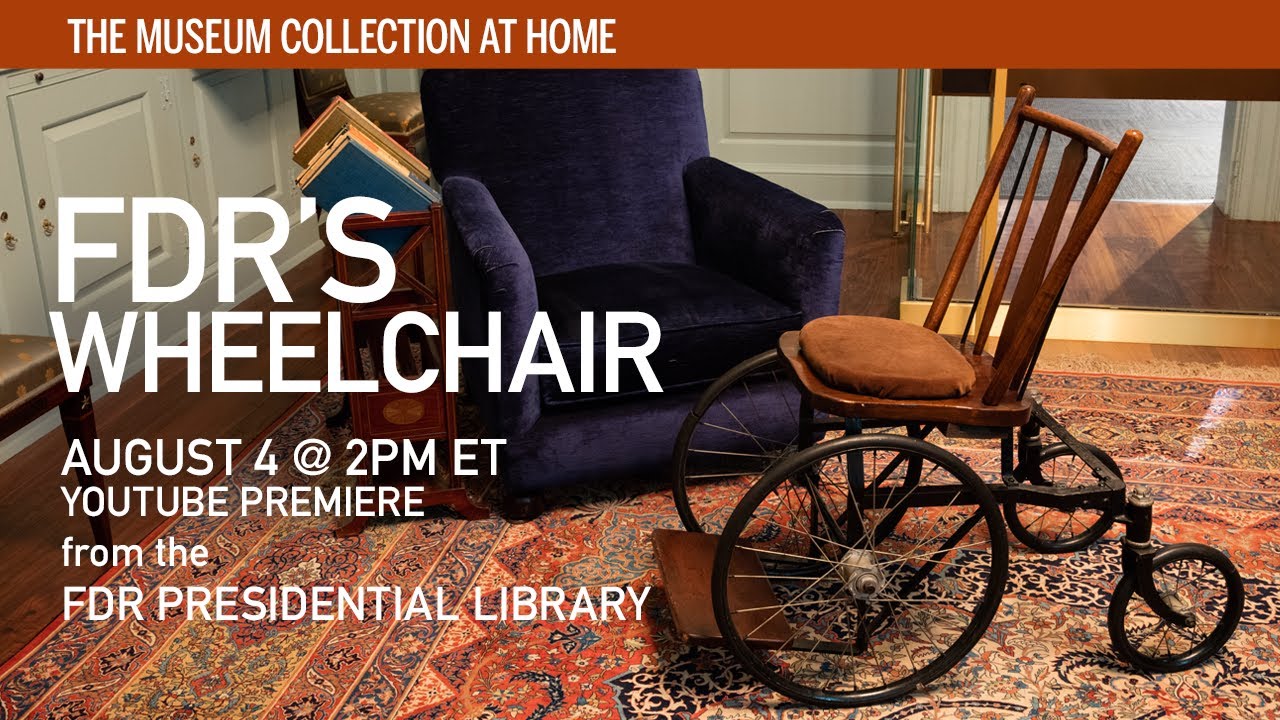This image, advertising a specific event, portrays a cozy living room scene with a detailed focus on FDR's wheelchair. At the top, there's a brown banner with white text reading "The Museum Collection at Home." The living room features a plush navy velvet chair, a decorative Oriental rug, and a small, well-stocked bookshelf with a few tomes on the top shelf. Dominating the foreground is an old-fashioned wheelchair, identified as Franklin D. Roosevelt's, characterized by its wooden frame and brown cushion, with two large wheels at the front and smaller wheels at the back. The text on the image announces a YouTube Premiere hosted by the FDR Presidential Library on August 4th at 2 p.m. Eastern Time, inviting viewers to explore museum collections from their homes.